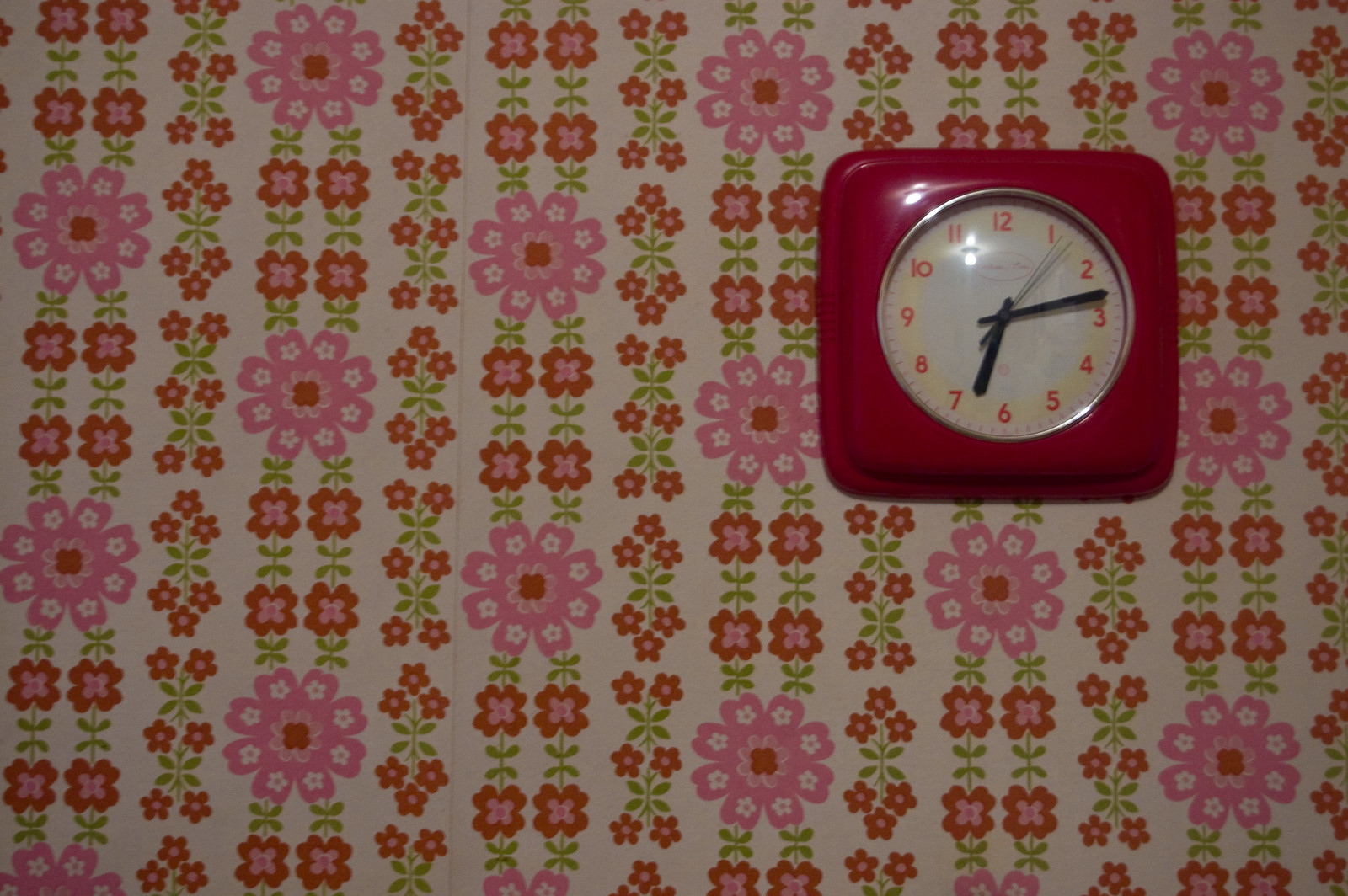In the cozy kitchen, the wall is adorned with elegant white wallpaper featuring a delicate pattern of pink and red flowers. Mounted on this floral backdrop is a striking clock, crafted in a radiant red square shape that exudes a glossy, wooden finish, reflecting light softly from an unidentified source in the room. The clock's design includes black hour and minute hands, a beige second hand, and bold red numbers marking each hour. Additionally, small red rectangles serve as minute markers, providing a detailed and functional aesthetic. The current time displayed on the clock is precisely 6:13.